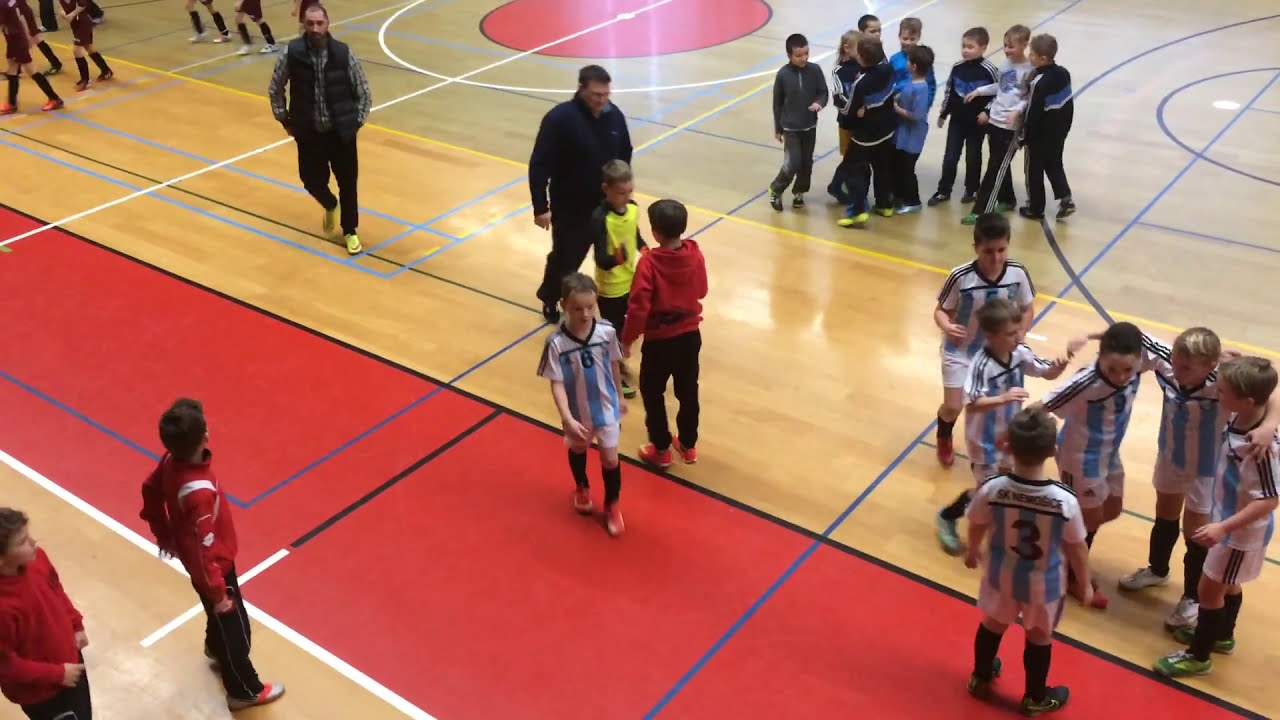The image captures a vibrant, bustling scene in an indoor basketball court gymnasium, taken from above. The floor is a mix of glossy light brown wood and red with various colored lines—white, black, blue, light blue, and yellow—marking different courts. In the bottom right corner, a group of boys in blue and white striped soccer uniforms huddle closely together. In contrast, the top right corner features another group of boys in sweatsuits, forming a similar cluster. Scattered around the gym are kids wearing a variety of attire, including black and blue jackets, red hoodies, and track pants. Adults, including one man in a plaid shirt with a black vest, meander amongst the groups, overseeing the activity. Farther into the background, other clusters of kids in magenta or crimson red soccer uniforms are also visible. The high-quality image is illuminated by bright indoor lighting, making every detail clear and distinct. Additionally, numbers such as 6, 3, and 9, along with possibly other digits, appear faintly visible on some of the kids' jerseys.